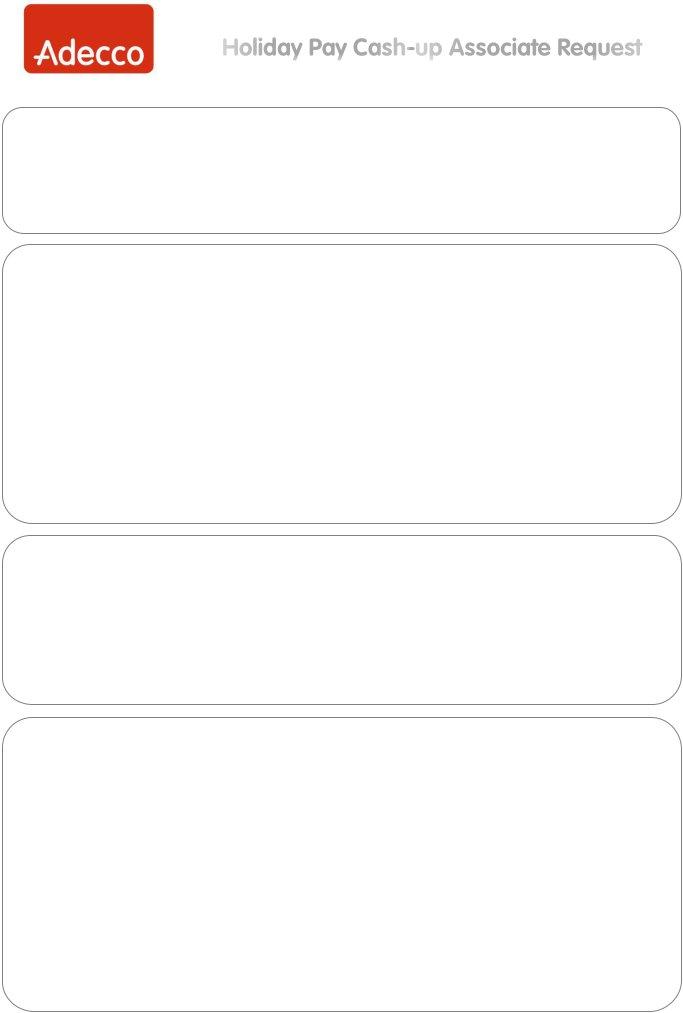This image showcases a mobile app interface in portrait orientation without clearly defined outside borders. At the top of the screen, there is a blank white header area containing some text and an input box. On the left side, there is a rectangular, vertically-oriented red button with rounded edges displaying the word "ADECO" in white lettering at the bottom.

The central section of the screen has a heading in grey text reading "Holiday Pay Cash Up Associate Request." Below this heading are four landscape-oriented rectangular boxes with rounded edges, positioned one below the other. Each box is outlined with a thin grey border and has slight spacing between them. The boxes vary in height but are uniform in length. The first box is the shortest, while the second box directly below it is tied for the tallest. The third box is slightly taller than the first, and the fourth box at the bottom matches the height of the second box.

The layout and design suggest that the app interface is related to requesting or managing holiday pay for associates, although the exact function and context remain unclear. The mix of text, input fields, and buttons indicates it may be part of a form or a request submission process.